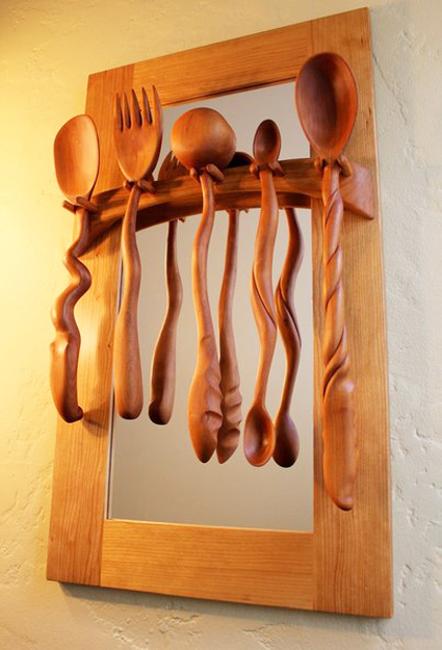This color photograph showcases a large, rectangular mirror with a thick, light beige, wooden frame that occupies most of the image. The mirror is mounted on an off-white, textured stucco wall. Illuminated from the left by what seems to be a tungsten light source, the scene features clear highlights and shadows enhancing the wooden textures.

Affixed near the top of the mirror's surface is a wooden rod that serves as a decorative utensil rack. This rod holds five large, artistically sculpted wooden utensils, each designed with unique, wavy handles and intricate engravings, emphasizing their ornamental nature rather than functional use. From left to right, the utensils include a wooden spoon with a wavy bottom, a wooden fork with a similarly wavy handle, a wooden ladle, a small double-ended spoon with spoons at both ends, and a long soup spoon with a rope-like pattern carved into its handle. Each utensil is hung between two small wooden knobs, contributing to the piece's artistic arrangement.

The entire setup, including the light and shadows, indicates that it is likely displayed in a residential interior, serving more as an artistic expression than practical kitchenware.